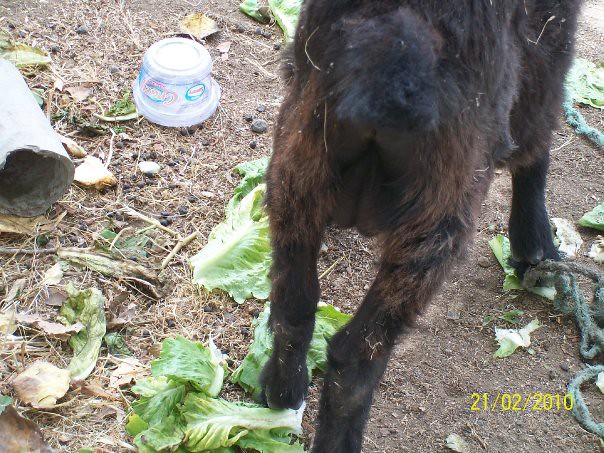In this whimsical farm scene photo captured on 21-02-2010, the focus is a goat seen from the rear, displaying its scraggly brown fur and slender black legs that end in hooves. The goat's hindquarters dominate the middle of the image, where even its udder or testicles are slightly noticeable. Scattered around on the dirt and dead foliage ground are green lettuce leaves and cabbage, suggestive of a recent feeding. An overturned plastic container, which might have once held food, rests in the top left corner, while a broken cement pipe lies nearby. Additionally, a blue, dirty rope can be seen cutting across the scene, adding to the farm’s rustic ambiance.